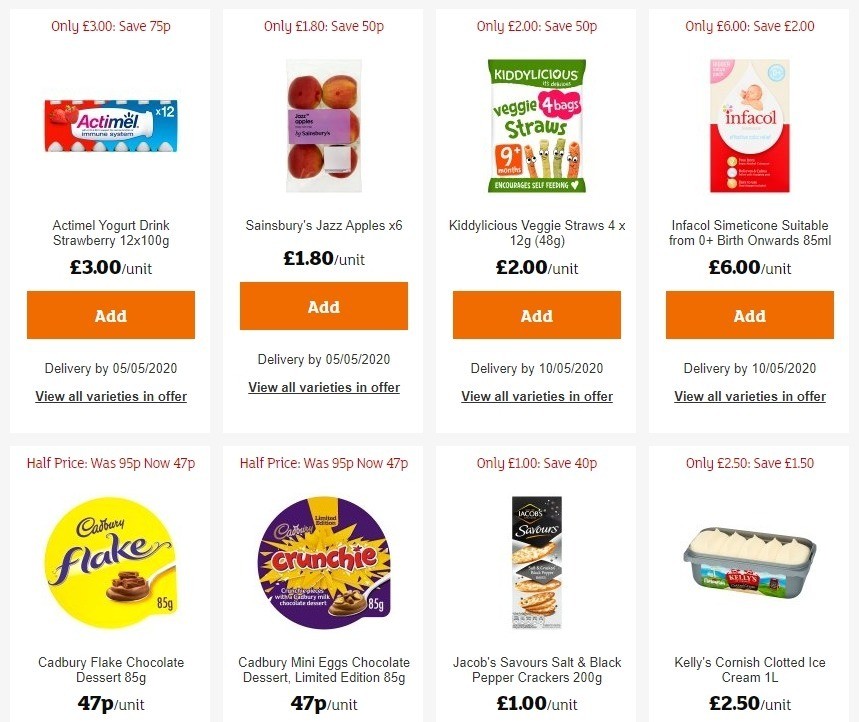This screenshot depicts a British online grocery shopping website, with prices listed in British pounds (£). The website showcases a selection of eight items, each accompanied by a clear picture, a detailed title, the price, and an orange "Add" button to add the item to the shopping cart. The displayed products appear to be primarily desserts, such as various flavors of ice cream and mini Cadbury chocolate desserts. One notable item in the list is Cadbury Flake Dessert. Another item includes Sandsbury Jazz Apples, indicating a broader selection that might extend beyond sweets alone.